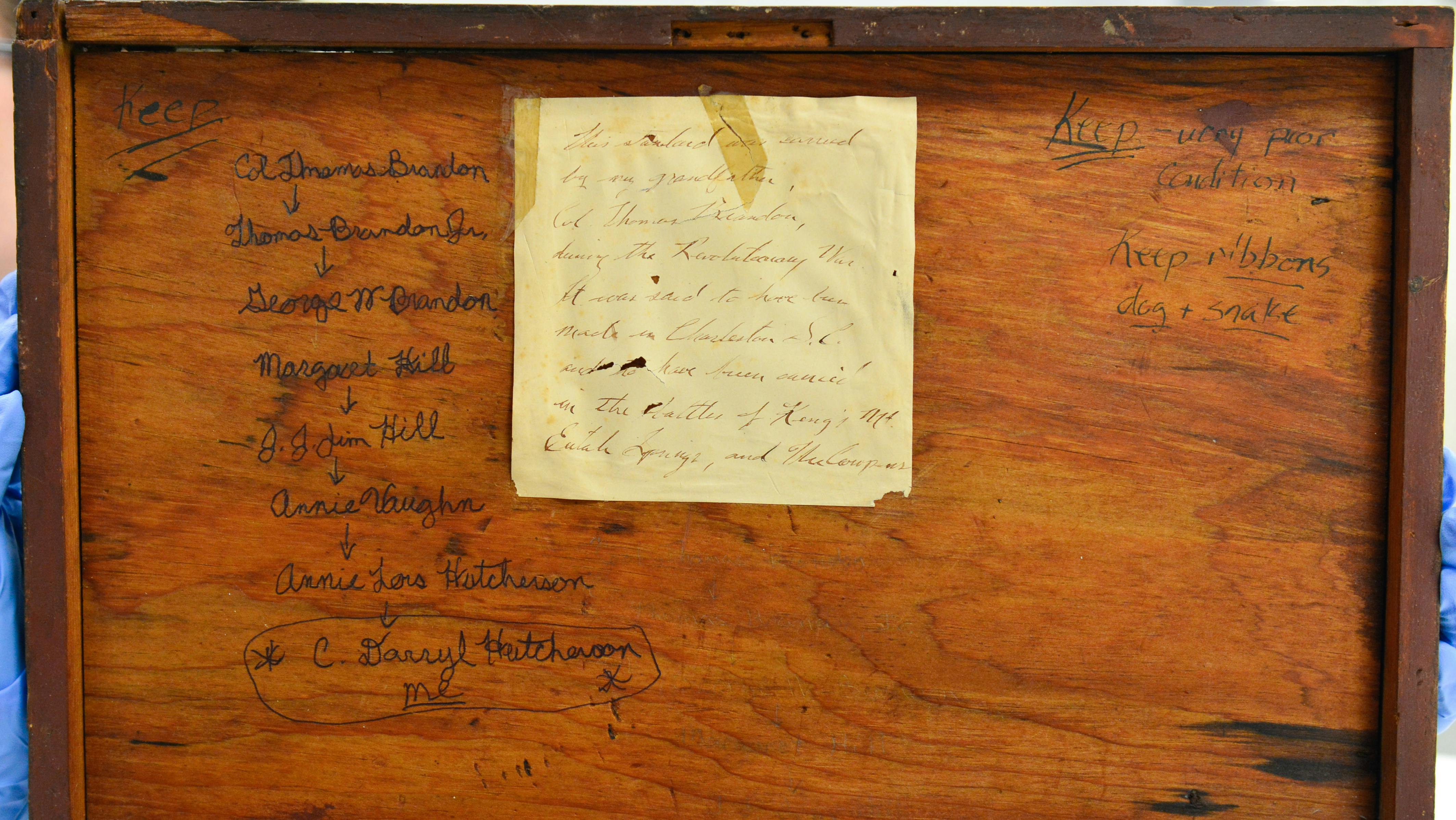The image depicts the underside of an old wooden desk that has seen a lot of wear and tear, with numerous names and notes written on it. The desk appears to have historical significance, as indicated by inscriptions and an old, lettered note attached to it with yellowed tape. This note, written in a calligraphy-like style, references Colonel Thomas Brandon, mentioned as having carried something during the Revolutionary War, possibly at notable battles such as Kings Mountain and Eufaula Springs. Additionally, various people’s names are scrawled across in markers, such as Thomas Brandon Jr., George N. Brandon, Margaret Hill, J.J., Jim Hill, Annie Vaughn, Annie Hutcherson, C. Darryl Hutcherson, and a few others. There's a recurring admonition to "keep," noted several times, along with cryptic references to "very poor condition," "ribbons," "dog," and "snake." The frame itself is a brown-painted wooden structure showing signs of severe fading, particularly in the upper left corner, with evidence of old screw or nail holes suggesting it might have once held a glass cover. The scene appears to be outdoors, with someone holding the desk—gloved hands are visible—with just a glimpse of their face.